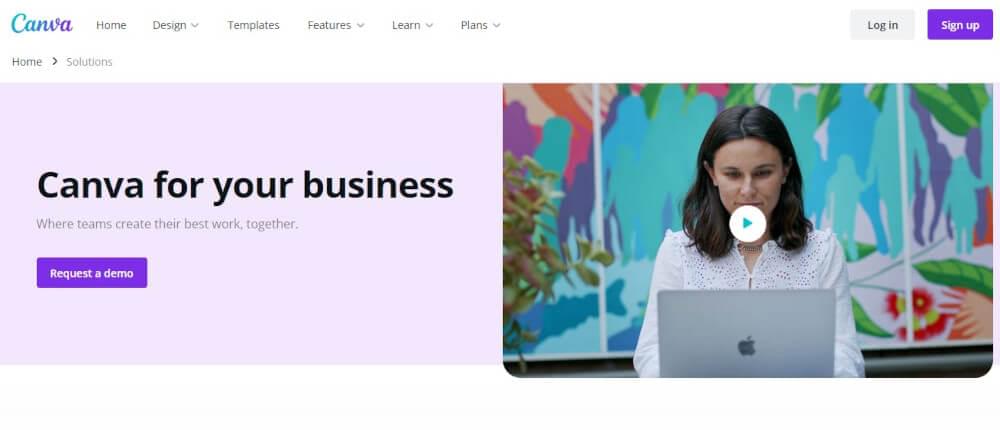This image is a screenshot of a webpage from Canva's website. At the very top, the Canva logo is displayed prominently, featuring a gradient: the letter 'C' is a teal color, 'A' and 'N' are blue, and 'VA' is purple. The navigation bar spans across the top with clickable options labeled Home, Design, Templates, Features, Learn, and Plans. To the far right, there are two buttons for user access: a gray 'Login' button and a purple 'Sign Up' button.

Directly under the Canva logo, the word "Home" is followed by an arrow pointing towards "Solutions." Beneath this, a purple banner stretches across the width of the webpage. On the right side of this banner, there is a vibrant, colorful image featuring a woman sitting and looking at an Apple MacBook laptop computer. This image is actually a video thumbnail, indicated by a white circle with a play-arrow icon in the center, suggesting the video can be played.

Within the purple banner, the text reads: "Canva for your business, where teams create their best work together." Below this, there is a purple box containing the text "Request a Demo."